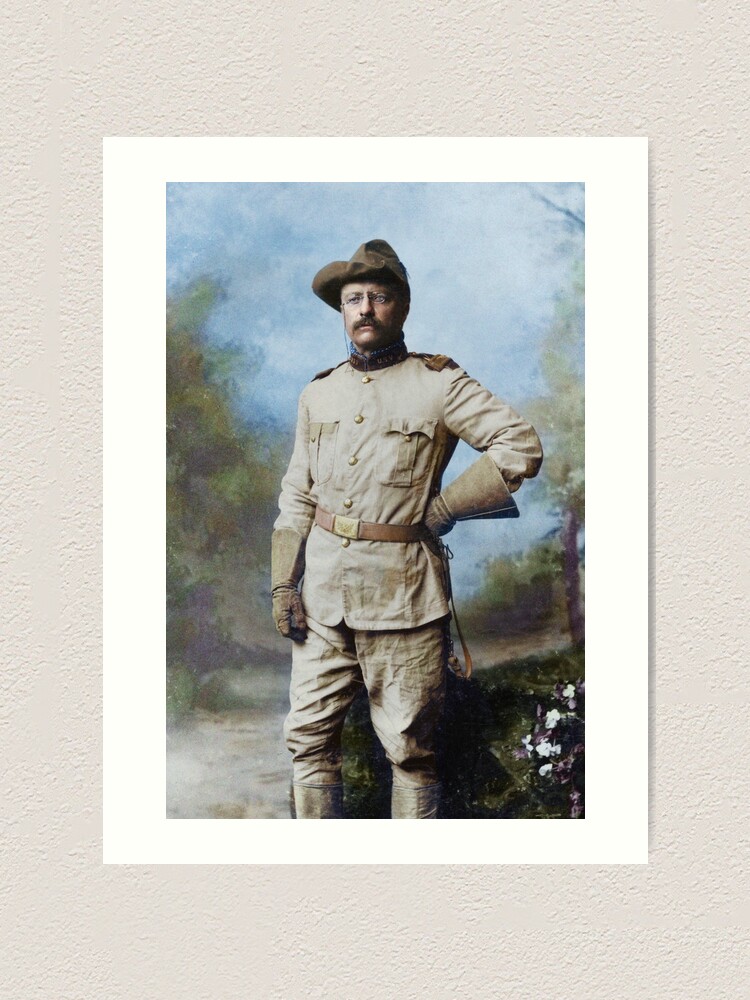The image is a digitized and colorized photograph of a man resembling Teddy Roosevelt, dressed in a vintage military or safari-style uniform. The man is standing in a posed stance with one hand resting on his waist and is wearing a brown hat, beige gloves reaching nearly to his elbows, a tan uniform, and a darker tan belt around his waist. His khaki pants are tucked into his boots, and he sports a handlebar mustache and spectacles. The background of the photograph is a painted depiction of a forest, characterized by its light and somewhat blurry quality. The photo is set within a white frame placed against a beige wall, adding to the old-fashioned, yet pristinely preserved nature of the image.